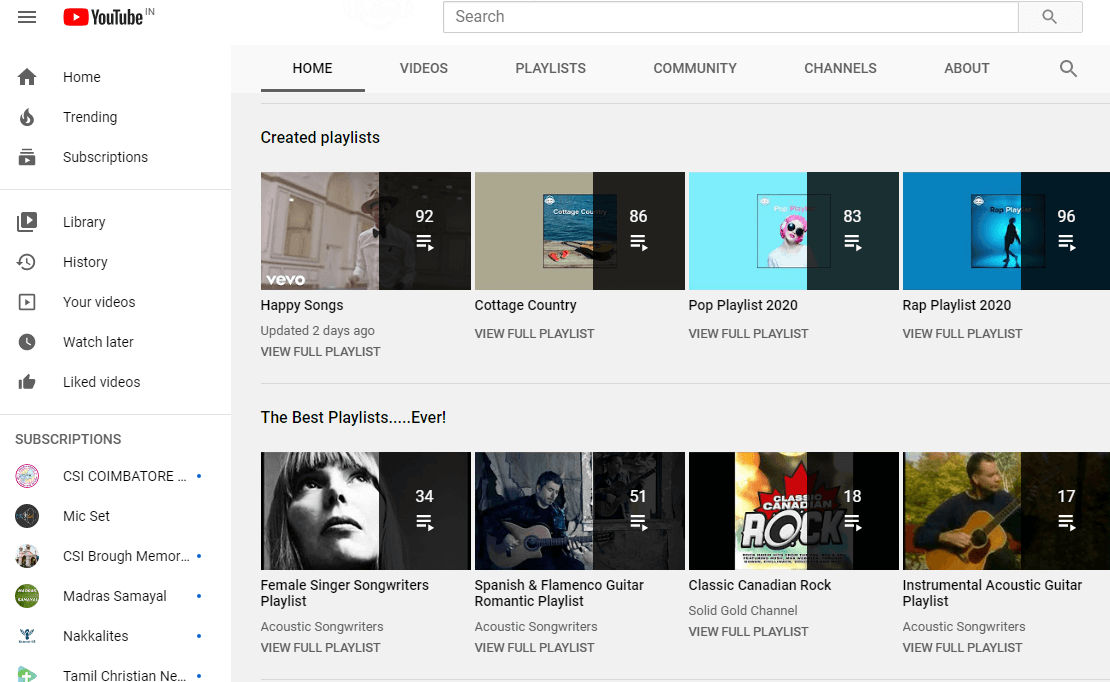This detailed image depicts the YouTube homepage interface. In the upper left-hand side, the YouTube logo and symbol are prominently displayed above a vertical navigation menu. This menu includes options in the following order: Home, Trending, and Subscriptions, followed by a gray separator line. Below the separator, the options continue with Library, History, Your Videos, Watch Later, and Liked Videos. Another gray separator line appears, after which the word Subscriptions is listed, showing the various channels the user is subscribed to.

On the main window area toward the right, the 'Home' section is selected. Below this, the interface presents several curated playlists, which are listed horizontally from left to right. The first playlist is titled 'Happy Songs,' followed by 'Cottage Country,' then 'Pop Playlist 2020,' and finally 'Rap Playlist 2020.' This setup provides a clear and organized overview of the YouTube interface and its menu options.